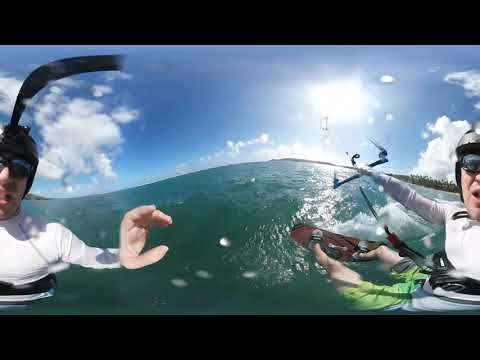The image depicts an outdoor scene with two men engaging in water sports, captured with a wide-angle, fisheye lens that creates a slightly distorted and cartoonish effect. Both men are wearing white long-sleeve swim gear and have black goggles. They are each holding onto a handle connected to a boat, indicating they are wakeboarding on a red and black wakeboard. The man on the left, who also appears on the right due to the fisheye distortion, is sporting green shorts and is waving his left hand towards the camera, creating a comically enlarged hand due to the lens distortion. The bright blue sky above is dotted with white clouds and a shining sun. Lush green trees and distant mangroves can be seen towards the right-hand side of the horizon. The water beneath them appears green, hinting at its depth. The playful expressions and the unique perspective of the image add a whimsical touch to this dynamic outdoor adventure.